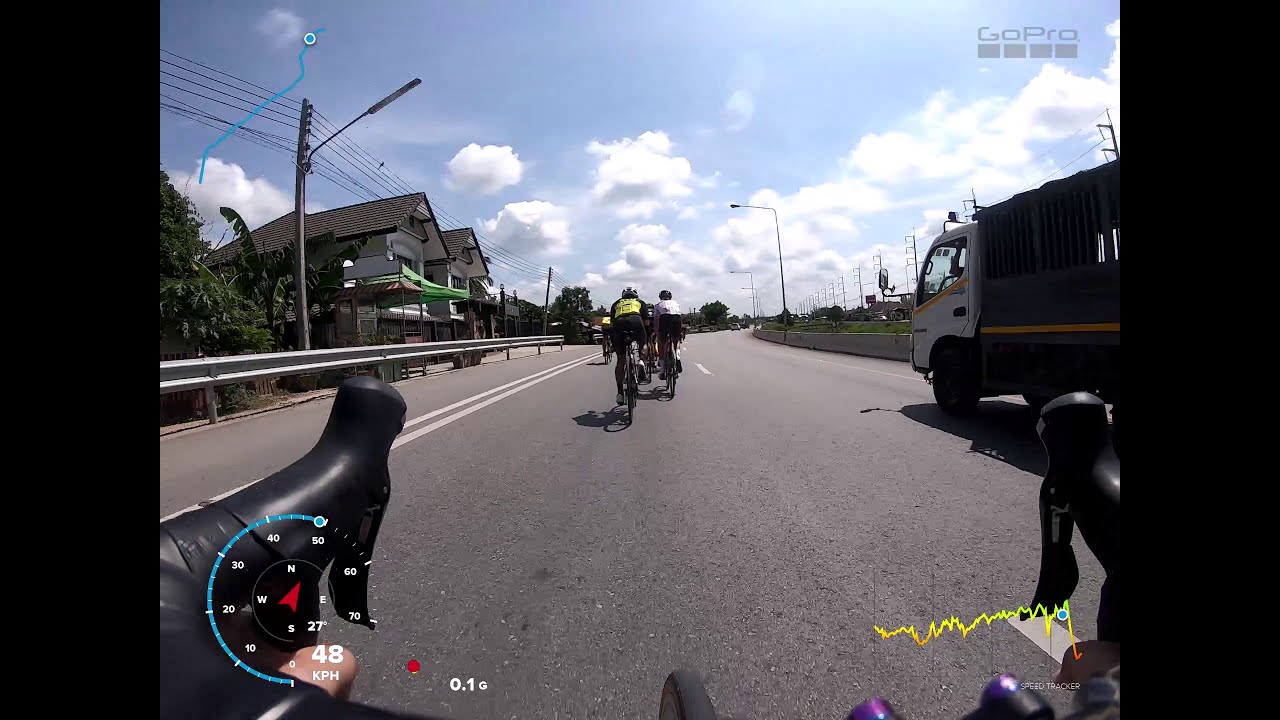This image captures a first-person perspective of a bicyclist riding on a road, as indicated by the "GoPro" label in the top right-hand corner. The scene unfolds with two black handlebars framing the bottom of the shot, and the faint thumb of the left hand visible on the left handlebar. The road stretches ahead, where several cyclists, their backs to the camera, pedal onward. One cyclist is wearing a yellow vest, and they appear distant and slightly blurry. 

To the right, a large white truck with a black back rolls by in the neighboring lane. On the left, a series of houses accompanied by a guardrail can be seen, along with telephone poles and street lights lining the path. Above, a partly cloudy sky with bright blue hues and fluffy white clouds adds a scenic backdrop.

Embedded in the screen are various dashboard elements: a speedometer in the bottom left showing the speed as 48 kph, with a red arrow indicating the direction as northeast. To the bottom right, there is a graph in green and yellow, possibly displaying heart rate or another variable, zigzagging sporadically. The viewer's position is marked in the left lane, bordered by a double line to the left and a dotted line to the right.